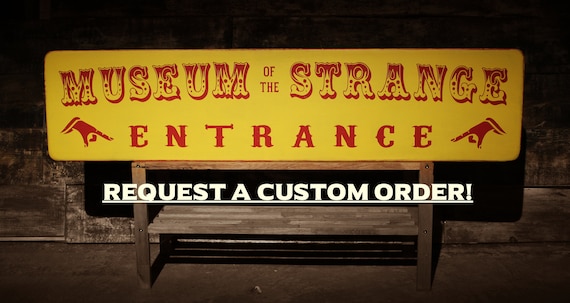In an old Western town setting, a photograph captures a rustic wooden bench set against a wooden-panel building. The ground is visibly dirty, adding to the Wild West ambiance. Positioned prominently on the bench is a bright yellow sign with deep red, old-fashioned carnival-style lettering announcing "Museum of the Strange." Below this title, the word "Entrance" is flanked by two red hands with index fingers pointing towards it. Additionally, the sign features a digitally overlaid request, "Request a Custom Order!" in bold white capital letters. The scene is vividly illuminated, with the camera's flash creating dramatic shadows, enhancing the authenticity of the setup. The image seems designed for a digital website banner, showcasing the bench and sign to highlight handcrafted, customizable products.